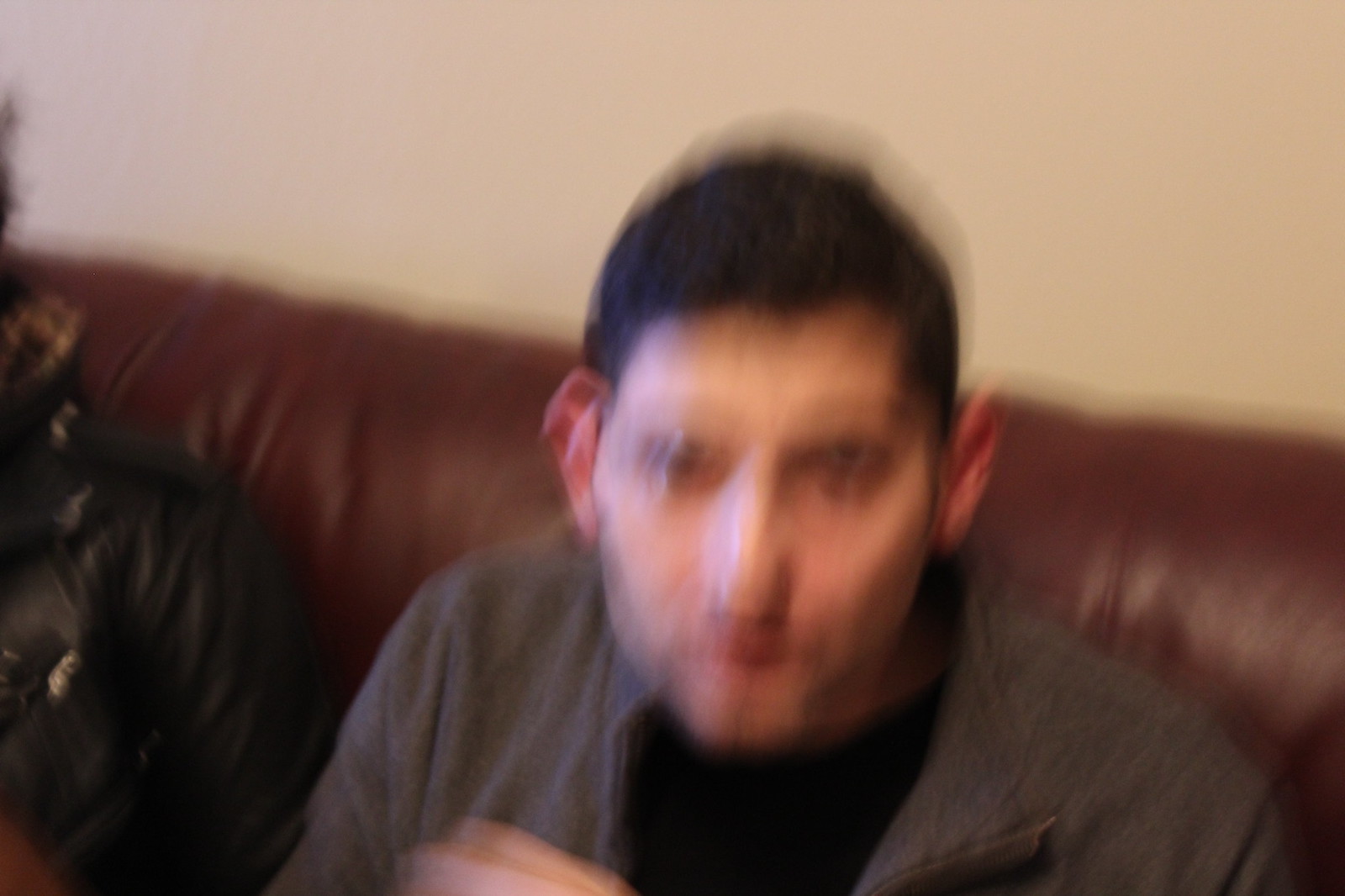The image is a blurred colour photograph of a white male seated on a dark brown leather couch against a plain, cream-colored wall. The man's short, dark hair has a slightly curly texture, and his fringe lines across his forehead. He has a few days' growth of facial hair and light five o'clock shadow around his beard and moustache. He is looking directly at the camera with an expressionless face, his red ears suggesting potential embarrassment or anger. He is dressed in a dark gray jacket or hoodie with a black shirt underneath. The blurring creates a double outline, particularly notable around his head. To his left on the couch, there appears to be a dark object with reflective gold elements, possibly a cushion or another person partly cropped out of the frame, though the details are obscured due to the blurring and cut-off nature of the image. His hand is visible at the bottom of the frame, slightly raised.